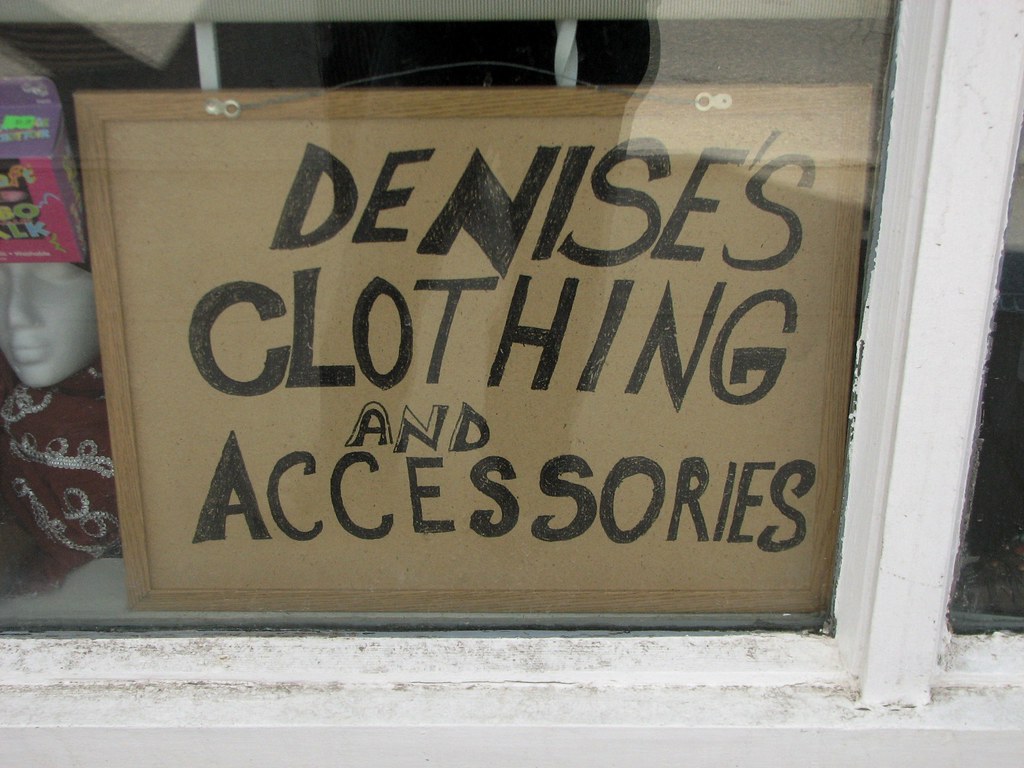This detailed photograph captures a close-up view of a sign affixed to a light brown wooden panel, prominently displaying the text "Denise's Clothing and Accessories" in bold black font. The scene is framed by a white window, creating a picturesque border. To the left of the sign, a white mannequin head is visible, elegantly adorned with silver jewelry placed below it. The reflection of the photographer can be faintly seen in the window, adding an element of mystery and human presence without revealing specific details of their appearance. The photo is taken in landscape orientation, enhancing the wide, immersive view of the storefront display.